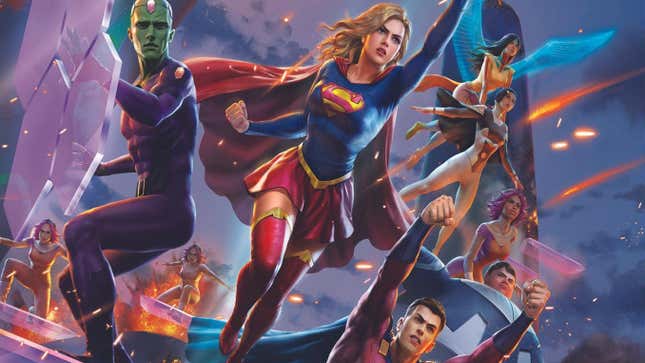This vibrant comic book panel features Supergirl, dressed in her iconic blue top with the distinctive red 'S' emblem, red miniskirt, and thigh-high red boots. She is captured in a dynamic pose, one arm extended upwards with her hand balled into a fist, as her red cape billows dramatically behind her. Surrounding her is an array of other superheroes and characters, each contributing to the bustling scene. To her left is a muscular figure in a tight purple outfit with a green face, possibly wielding a glass shield. To the right, a variety of superheroes, both male and female, in colorful outfits, are either flying, standing, or gesturing with hands raised, creating a sense of readiness for battle. The backdrop is a muted dark sky, streaked with hues of orange, yellow, and green, interspersed with fiery sparks and glowing lights, lending an intense and chaotic atmosphere to the scene.